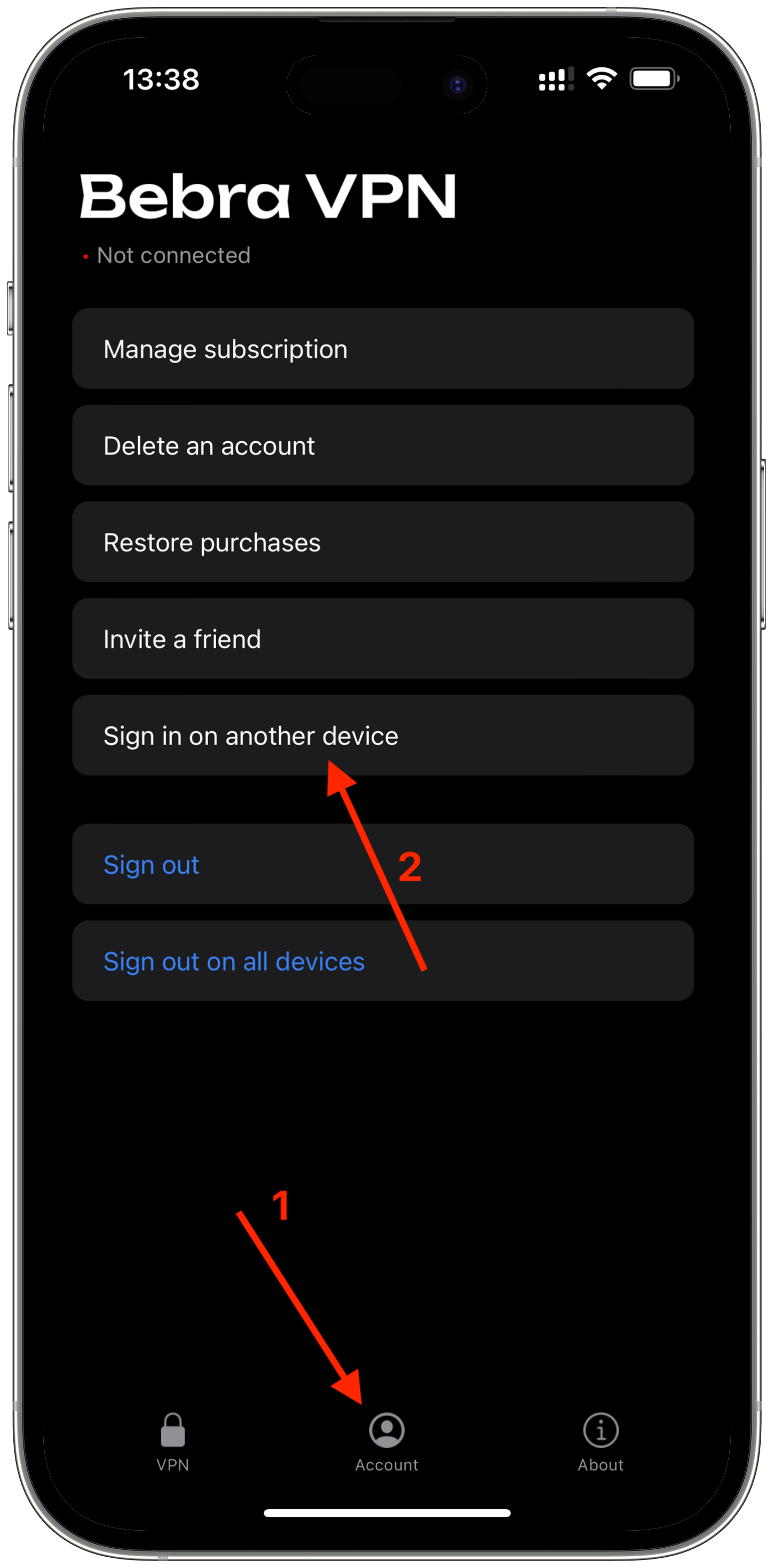The image displays a simulated cell phone screen with a silver bezel and silver buttons on the side. The phone screen has a black background, with the top displaying the time "13:38" in white text. Alongside the time, icons for Wi-Fi, battery, and a label "BEBRA VPN" (in white text) are visible. A red asterisk next to the label indicates that the VPN is "not connected."

Below this top section, there are multiple dark gray boxes with white text, which read as follows:
- Manage subscription
- Delete account
- Restore purchases
- Invite a friend
- Sign in on another device (this box includes a red arrow pointing up with a number "2" beside it)
- Sign out (in blue font)
- Sign on all devices (in blue font)

Further down the screen, there is a black section featuring another red arrow, numbered "1," pointing to a gray and white circle icon resembling a head and shoulders silhouette. The gray text label under this icon reads "Account," flanked by a thin white line. On either side of the person icon are two additional icons: a padlock labeled "VPN" and an "i" in a gray circle labeled "About."

The image quality is clear, and there are no other objects of note present.